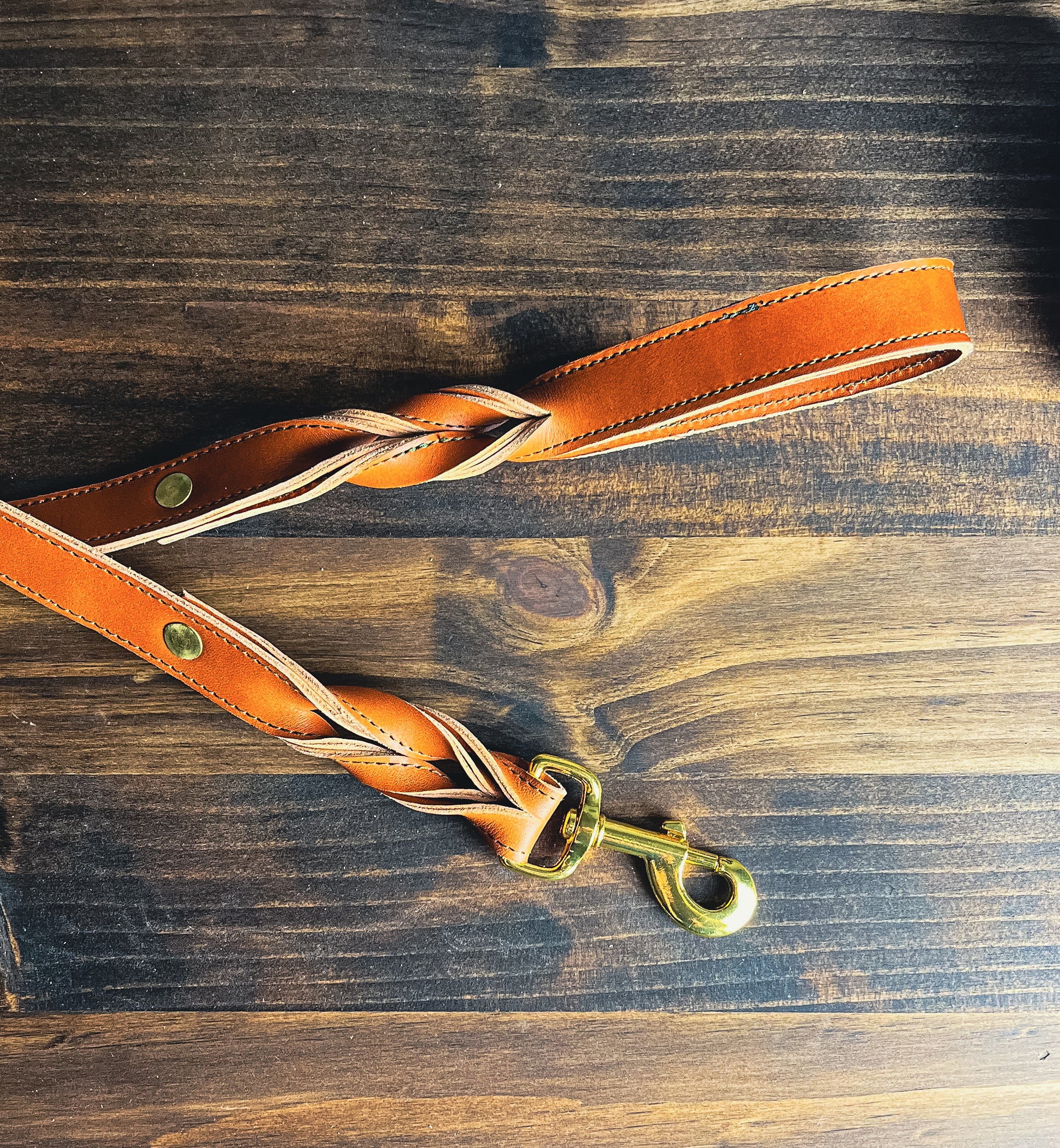This color photograph, measuring eight inches by eight inches, depicts an orange leather dog leash intricately laid out on a wooden table composed of several planks with visible knots and grain patterns. The leash, made from orangish-brown leather with stylized triangular detailing and a combination of tan and black accents, features prominent stitching along its edges. The leash is folded over itself, creating a series of curls and twists, and includes a looped handle on the upper right side. The brass clip, located lower on the image, is golden in color and designed to open by pressing a small lever. The wooden table beneath the leash consists of planks varying in color from light to dark brown, with the darker hues becoming more pronounced towards the top of the image, adding depth and contrast to the photograph. Various portions of the leash are visible: the handle emerges from the left side, while another part extends vertically toward the bottom, making a slight arc before exiting the frame.